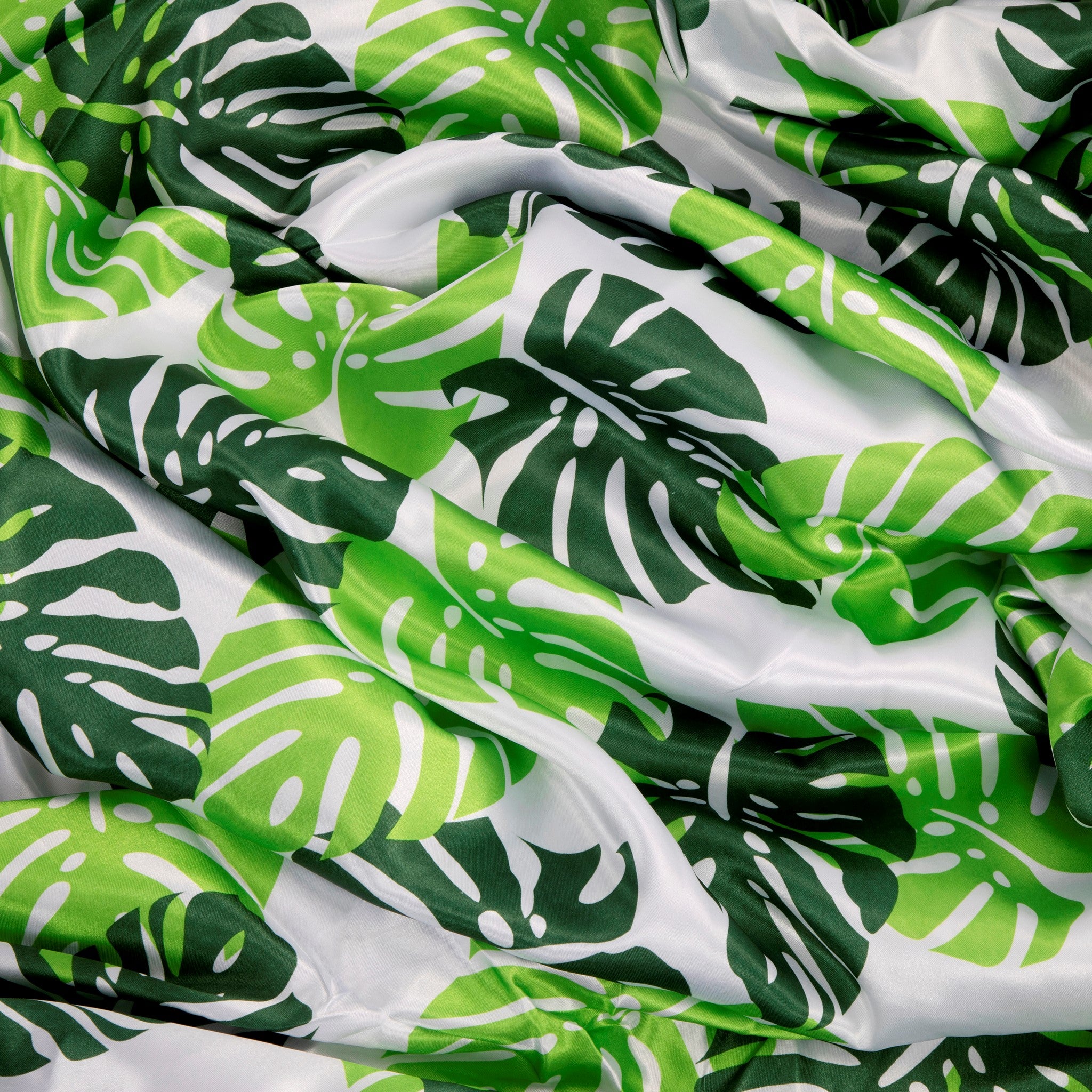This close-up image showcases a piece of shiny, satin-like fabric, which could be part of either a scarf, a satin blanket, or a clothing item. The material, characterized by its smooth and wavy texture, is bunched up in places, giving it a dynamic appearance. The fabric has a white base, which occupies the entire image, contrasting beautifully with a repeating pattern of large tropical leaves. These leaves, which are palm-shaped with heart-like tops and pointed bottoms, feature alternating tones of green. Some leaves are a bright, neon or lime green, while others are a rich, luscious dark green, possibly reminiscent of emerald or forest green. The interplay of these two shades against the shiny white background adds to the vibrant, elegant aesthetic of the fabric.